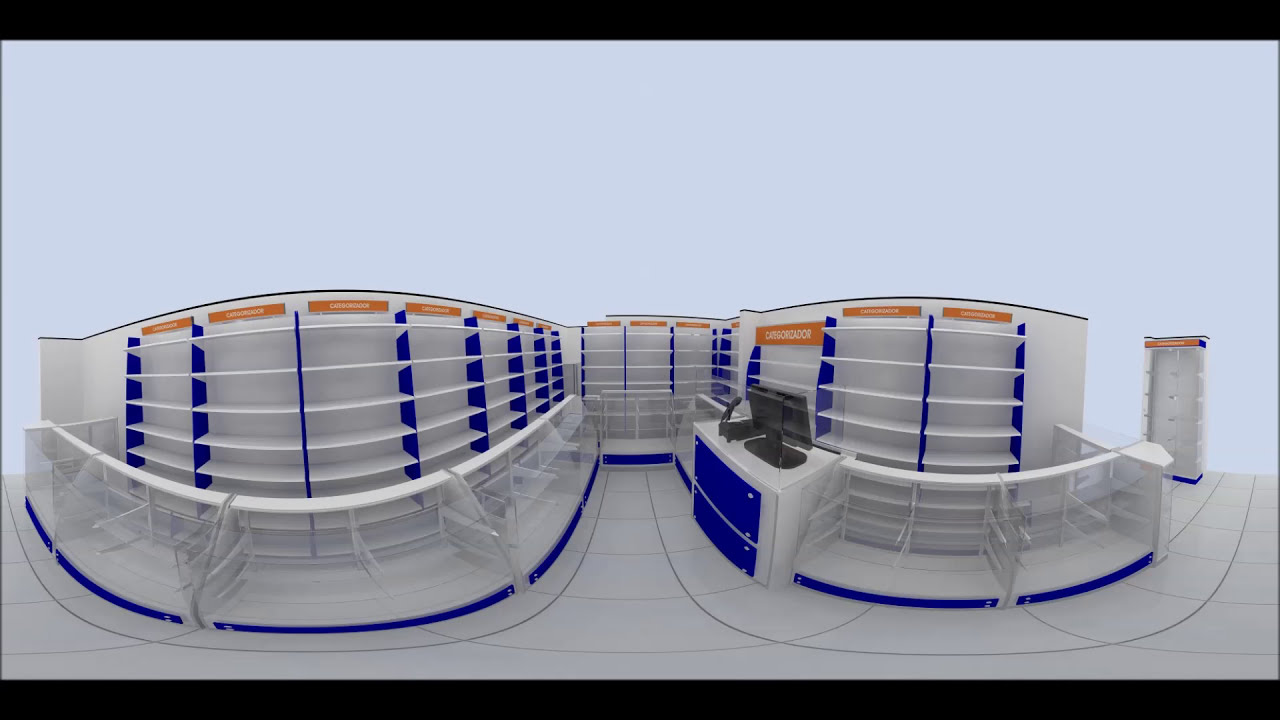The image depicts a digitally created mock-up of a storefront interior, likely designed for virtual reality training or visualization purposes. The scene is characterized by several clear, empty shelving units devoid of products, arranged in five levels with bright blue dividers between them. At the top of each shelf are orange labels with white lettering, although the text is unreadable. The background is a light blue, creating a stark contrast with the primarily white and blue color scheme that dominates the scene. In the lower right-hand corner, a white counter with blue paneling hosts a black computer monitor on a stand, suggesting a point-of-sale area. The floor features a square-tiled pattern, adding to the overall minimalist and somewhat sterile aesthetic. The absence of people or other items contributes to the impression of an unoccupied or preparatory training environment.